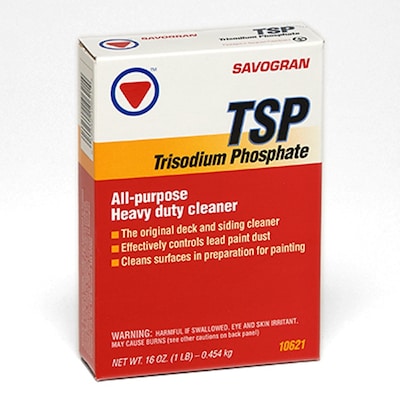This is a detailed color photograph of a product box for Trisodium Phosphate, commonly known as TSP. The box resembles the shape of a cereal box but serves an entirely different purpose. The top section of the box features a white border with the brand name "SavoGran" in red letters on the upper right corner. Beside it on the upper left, there is a logo consisting of a red triangle encircled by a blue ring. Beneath the brand name, large black letters spell out "TSP," with "Trisodium Phosphate" written in smaller black text just below, set against a light orange or yellow band.

The bottom portion, covering approximately 60% of the box, is red. Prominently displayed in this section, the white text reads "All Purpose Heavy Duty Cleaner." Below this, three orange square bullet points detail the product's features: "The original deck and siding cleaner," "effectively controls lead paint dust," and "cleans surfaces and prepares them for painting." Further down, in small white text, are warnings and the net weight of the product, specified as 16 ounces.